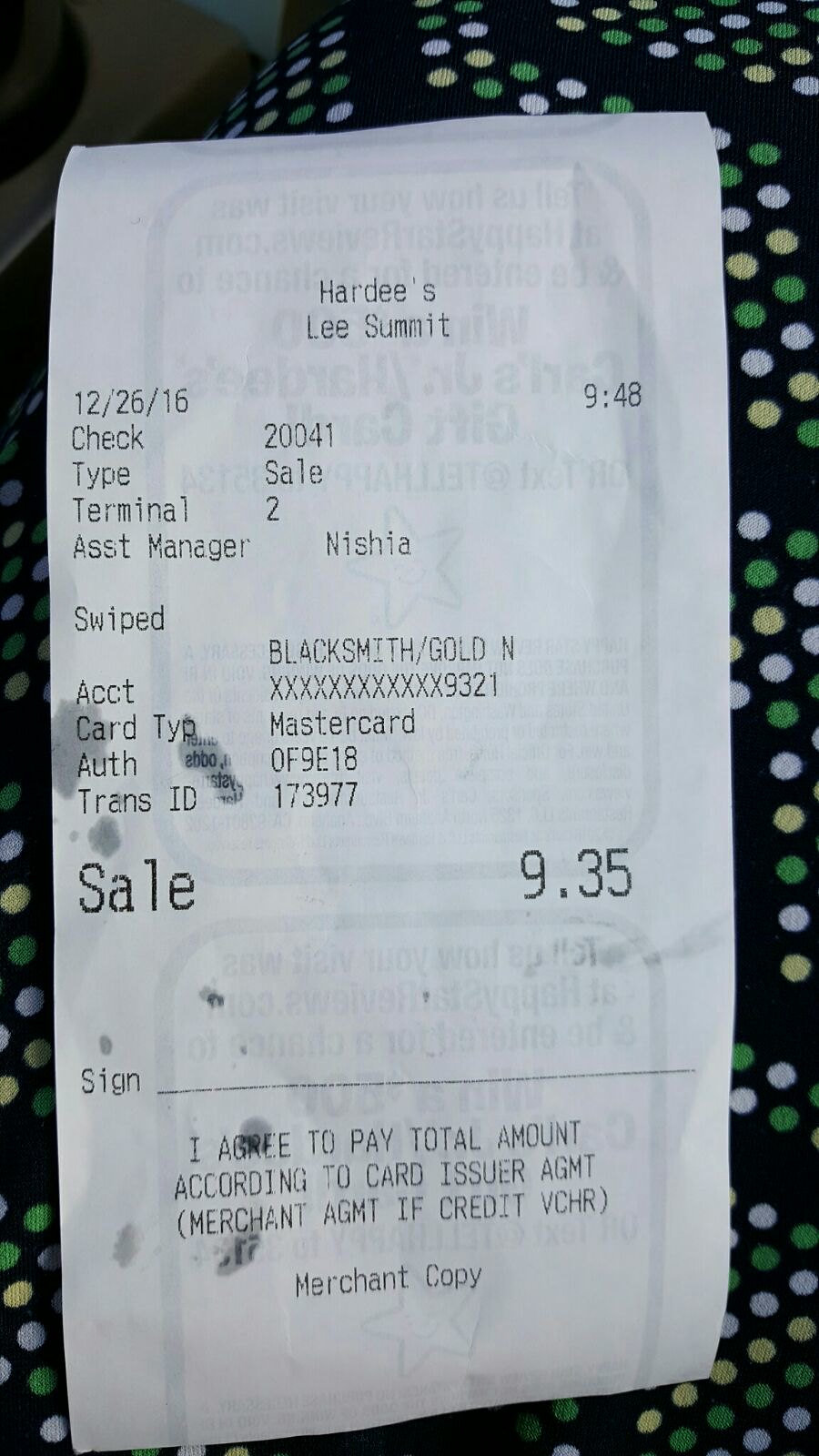A high-resolution photograph showcases a white paper receipt resting on a soft, black surface adorned with green, yellow, and white polka dots. The receipt bears the date December 26, 2016, and is issued by a Hardee's in Lee's Summit. The receipt details include a check number, 20041, being processed through terminal 2. The transaction involved a MasterCard and the assistant manager who handled it. The total sale amount is listed as $9.35. The receipt features a signature line at the bottom, accompanied by the text, "I agree to pay total amount according to card issuer agreement." It is clearly marked as the "Merchant Copy" at the bottom.